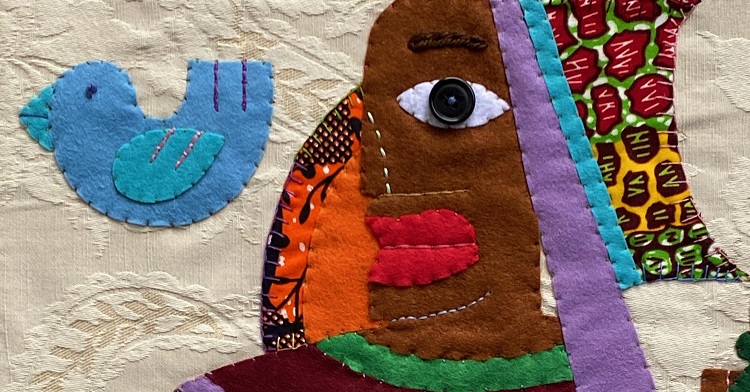A detailed piece of needlework displayed on a white damask background fabric with embroidered floral etchings. On the left-hand side, there is an appliquéd felt bird with a blue body curved gracefully, adorned with a lighter blue wing, a lighter blue beak, and an embroidered eye. More towards the center, an abstract face is crafted from various fabrics. This face features a brown area with a black button eye surrounded by white fabric, a red fabric forming the lips, and an embroidered eyebrow above. An orange piece of fabric situated on a black checkered pattern sits behind the face. Below the face, a green stripe swirls downward like part of a shirt. Adjacent to this abstract face, a series of colorful stripes—from purple to blue—lead to an intricate and vibrant patch. This patch includes red and black spots, a green and white background, and areas with letters like "VKI" and "VVI," contributing to the piece's complex, colorful design that evokes imagery of a gaily dressed, abstract figure, reminiscent of African-American culture in a lively hat and bonnet. The overall composition resembles a playful mural blending whimsy and abstraction.